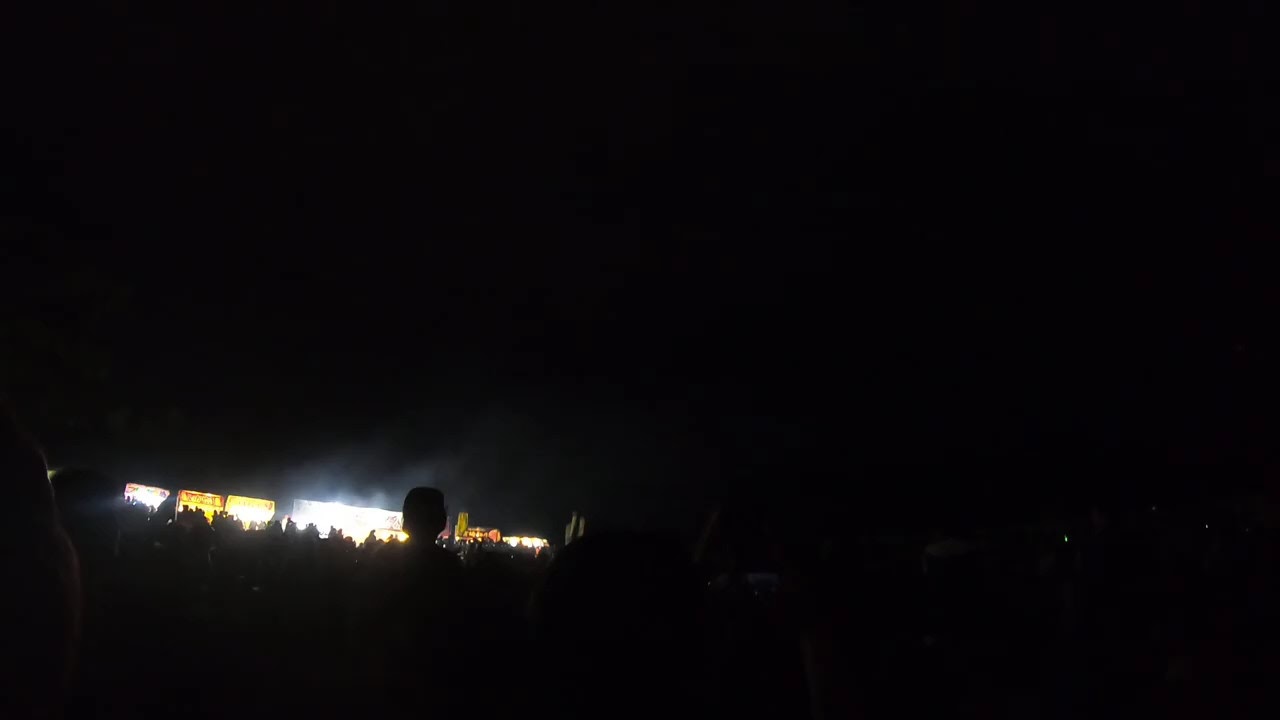The image is predominantly black, with minimal visibility except for a narrow stripe of white light in the bottom left corner. This illumination seems to be coming from an open door or large window, suggesting it originates from outside and casts light into an otherwise dark interior. Within this stripe of light, silhouettes of multiple people can be seen standing, possibly indicating a gathering. The left side of the image also reveals a group of people whose heads are discernible, hinting at a crowded space. Additionally, there are signs or screens visible in the background, which could imply that this scene is taking place during a concert or some event. The darkness intensifies towards the center and right portion of the picture, making it challenging to distinguish any further details.